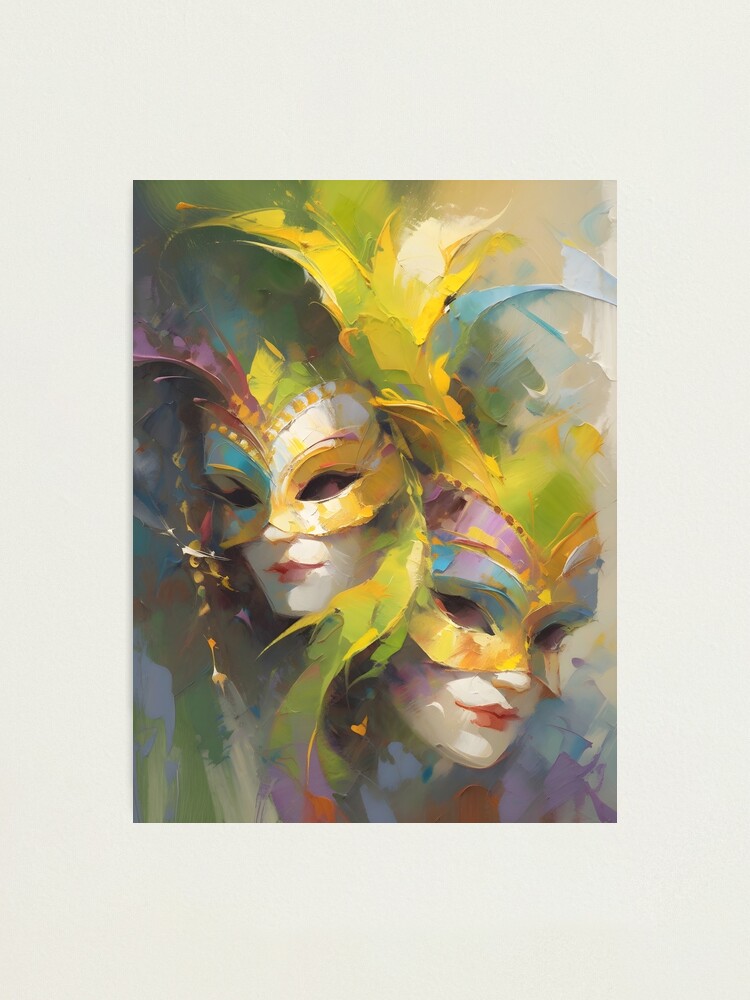This vibrant and detailed painting, potentially using oil or acrylic mediums, showcases two nearly identical, pale-white faces with bright red lipstick, each exquisitely adorned with brightly colored masks and extravagant feathers. The masks, typical of New Orleans Mardi Gras, cover only the eyes and feature a palette of gold, blue, yellow, turquoise, purple, and green, seamlessly blending into the abstract and pastel-toned background. The background itself transitions smoothly between shades of brown, green, blue, tan, and purple. The figures stand centrally within the portrait-oriented artwork, which is either bordered by a thin gray frame or set against a wall without a visible frame. The faces, one slightly lower and turned to the left and the other slightly to the right, both exhibit a mysterious and theatrical essence. Decorative elements such as yellow beading around the eyes and an array of feathers—ranging in color from pink to yellow to green—further enhance the whimsical, colorful, and carnival atmosphere of the scene.